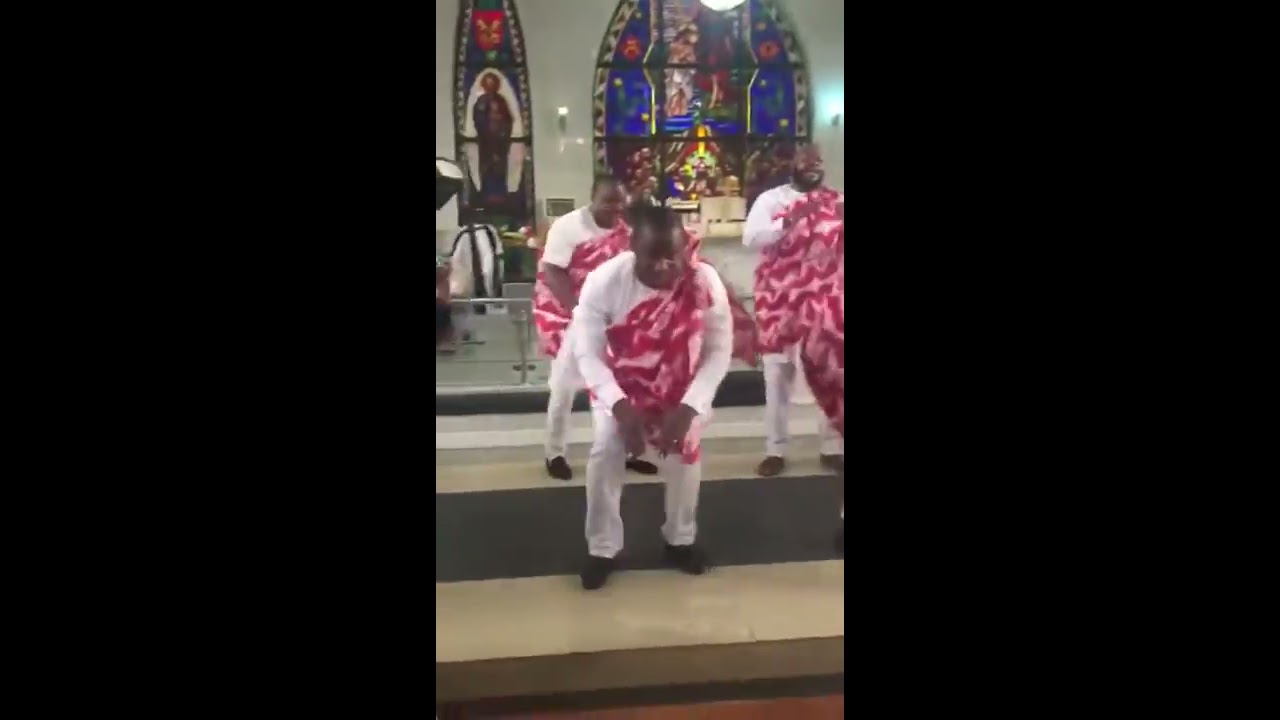In this detailed image, we see three Black men adorned in matching traditional attire, standing and dancing on a two-tiered stage at the front of a church. Each man wears a white long-sleeved shirt, white pants, and black shoes. Draped diagonally from their left shoulders is a vibrant sash in hues of pink, purple, and white, reminiscent of a ceremonial garment. The man on the lower step has his hands on his knees, while the two men on the higher step appear to be rising from this pose, capturing them mid-motion in what seems to be a coordinated dance.

The backdrop of this lively scene is defined by the church's signature architectural elements. Dominating the white wall is a large stained-glass window in an arch shape, featuring intricate, colorful designs and multiple figures. To its left, there is a smaller stained-glass window depicting a single person. Both windows are vibrantly illuminated, enhancing the ecclesiastical atmosphere. Flanking the large stained-glass window are light arches, perhaps suggesting torches or other forms of lighting, contributing to the sacred ambiance. Below the stage, a gray railing frames the dancers, while the floor beneath them sports a striped pattern in shades of black and dark brown. The photograph itself is framed against a black background, emphasizing the vivid activity and rich detail within the church setting.